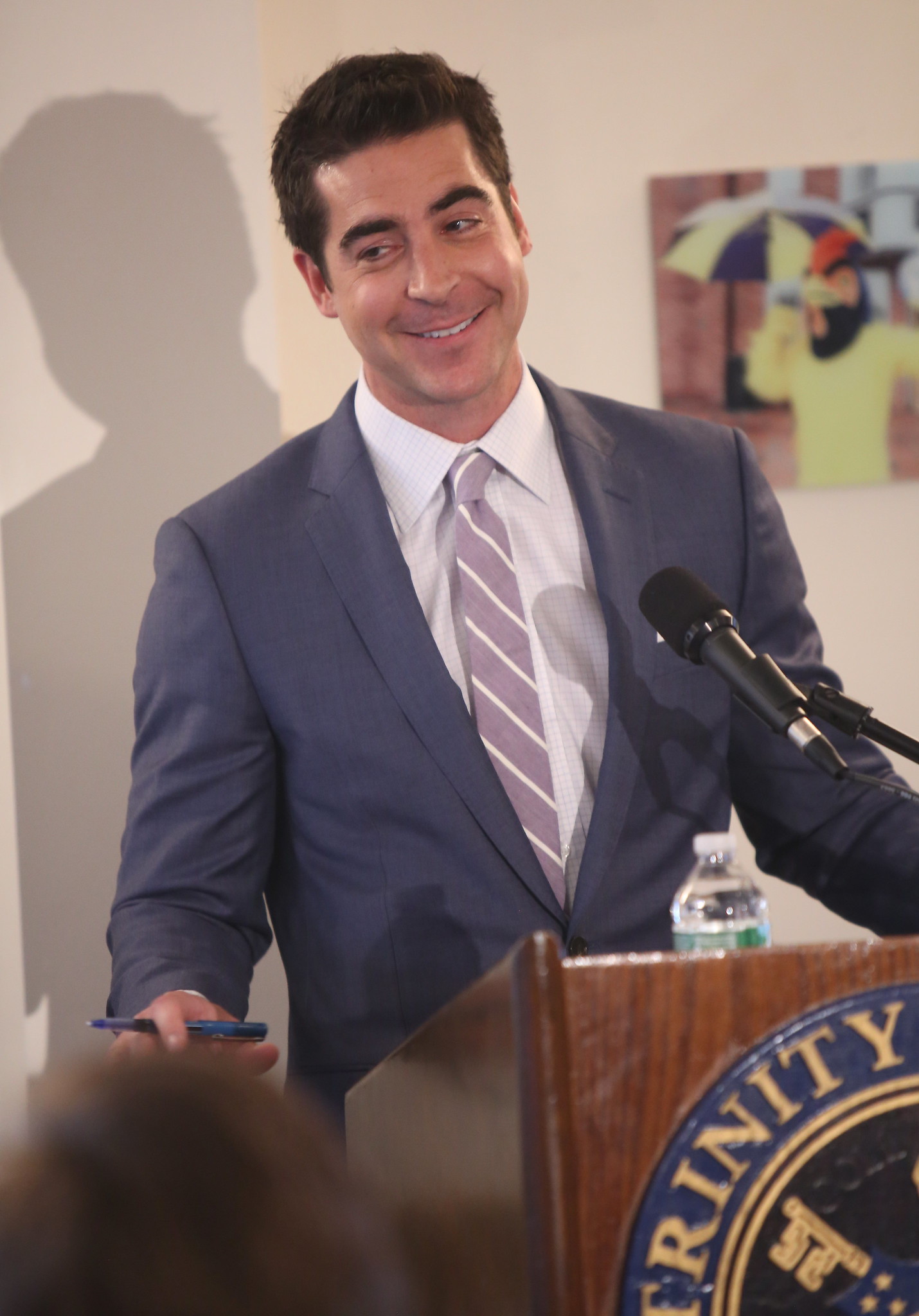This photograph features a white-skinned man standing behind a brown wooden podium adorned with a partially visible circular blue and gold logo, reading "Trinity" in gold letters with a key emblem. The podium is equipped with a wired black microphone and a water bottle with a green label. The man, dressed in a mid-blue blazer, white button-down shirt, and a gray and white striped tie, is smiling and looking slightly to his left, his shadow cast on the off-white wall behind him. He holds a blue marker pen in his right hand. The wall displays a peculiar picture of a person wearing a red beret and a yellow shirt, possibly in a costume, and holding a black and yellow umbrella.